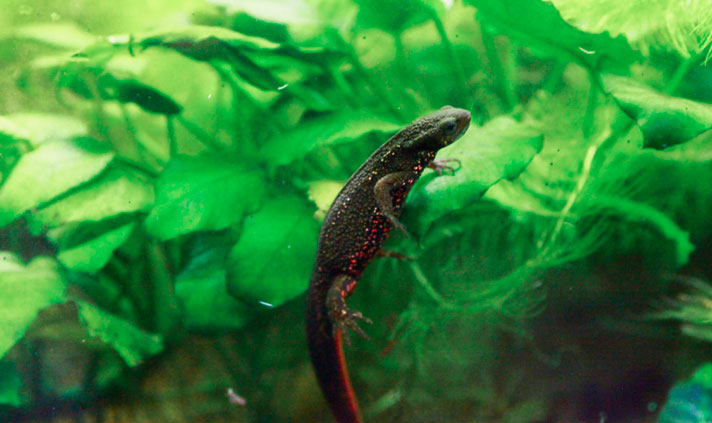This image captures a small, lizard-like reptile perched on a vibrant, green aquatic plant. The lizard is predominantly black or very dark green and is adorned with numerous bright red and yellow spots along its belly. The underside of its long tail features a distinct red stripe. Although the very tip of its tail is cut off in the frame, the focus is sharply on the lizard, which sits centrally on the plant, suggesting it is either climbing or walking. You can see its small head, thick neck, and one of its eyes clearly, with its legs and feet appearing in motion. The background, comprised entirely of green plant matter, is artistically blurred due to a high depth of field, emphasizing the lizard against a soft, diffuse background. The image is clear and well-composed, with a noticeable contrast that draws attention to the reptile against the lush greenery.